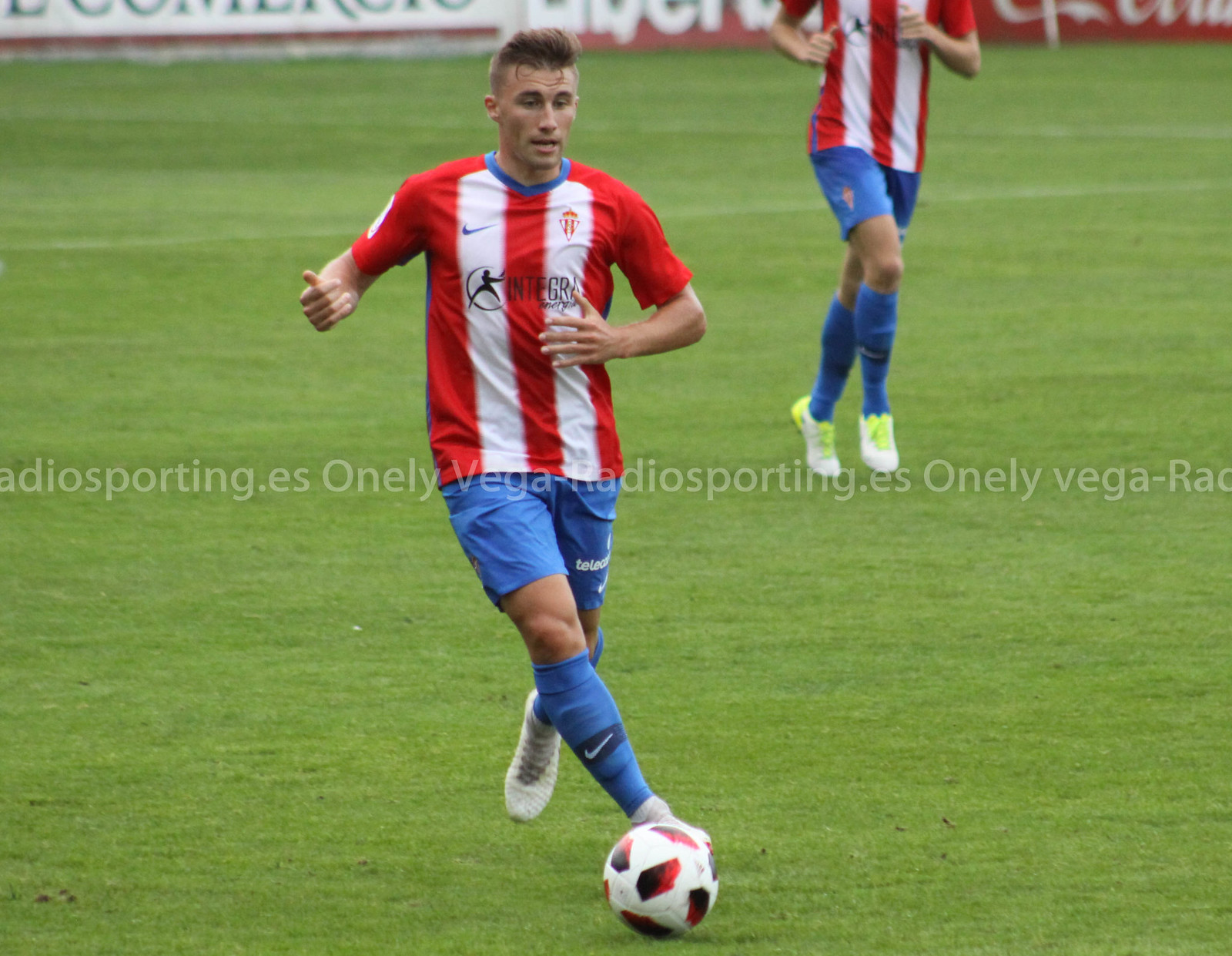In this photograph, two soccer players are captured in action on a green pitch. Both players are dressed in red and white vertically striped tops with blue collars, paired with light blue shorts and socks, and white shoes. The first player, centrally positioned, is actively kicking a white soccer ball adorned with red and black markings. Notably, this player lacks the visibility of their head or face as the image cuts off at the shoulders. The second player, positioned towards the upper right-hand side, is partially visible and appears to be running. This player also has the same uniform and features bright green laces on their white shoes. In the background, there are advertisement boards in red, white, and black colors, though they are partially cut off and illegible. Additionally, there is some white text across the middle of the image, written in a different language, further adding to the scene's dynamic ambiance.